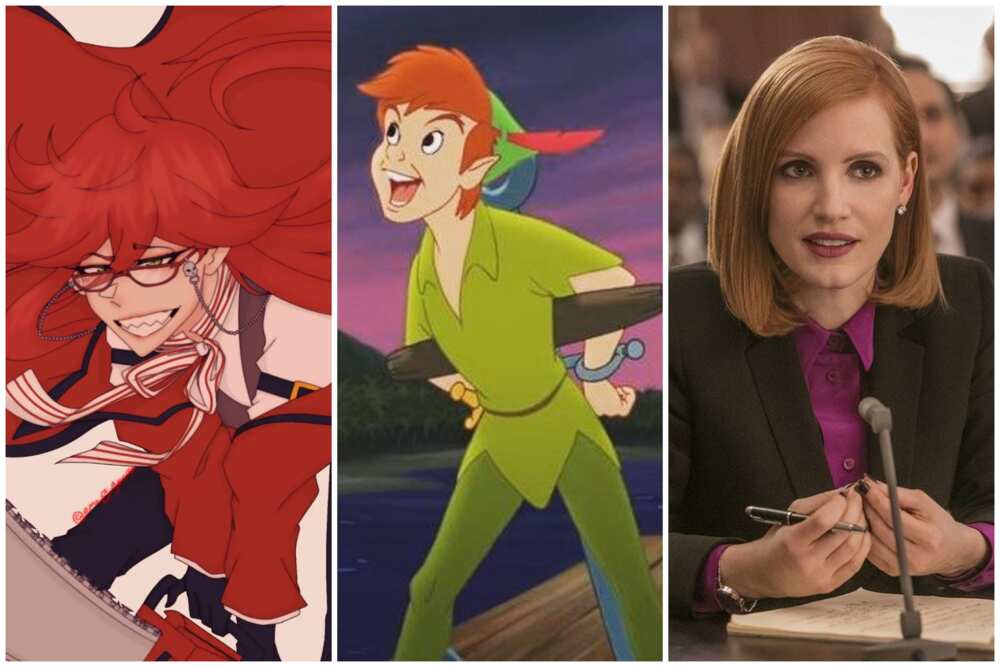The image consists of three vertically aligned rectangular pictures, separated by a vertical white line. The left picture is a close-up cartoon image of a woman with vibrant red hair that is flying out behind her. She is smiling, revealing her teeth, and wearing small red reading glasses with a chain. She has on red pants, a white top, and a red and white ribbon tied around her neck. The middle image features Peter Pan, the cartoon character, with brown hair and a notable green hat adorned with a red feather. He is dressed in a green outfit and is shown shouting upwards towards the left, with his hands behind his back, appearing to be handcuffed to a board. The right picture is of an actress, possibly Bryce Dallas Howard, with short, shoulder-length reddish-brown hair parted to one side. She is wearing a black suit jacket over a purple button-down shirt and has black nail polish. She is seated in front of a microphone, holding a pen with her fingers together and smiling slightly.